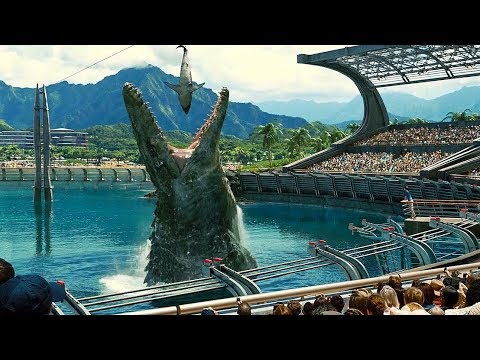The image captures a dramatic scene from the movie "Jurassic World," one of the latest franchises in the Jurassic Park series. In the center of the image, a giant prehistoric sea creature, resembling a massive crocodile, is seen leaping out of a man-made pool or lagoon with its jaws wide open, ready to devour a shark hanging from a cable. This scene, reminiscent of a SeaWorld performance, showcases a large crowd of spectators seated in modern, curved grandstands that surround the pool. The stands are filled with people, adding to the sense of awe and excitement. In the backdrop, the lush greenery of a tropical island is visible, complete with tall, majestic mountains and clouds hovering above, capturing the essence of the exotic and thrilling environment that is Jurassic World.